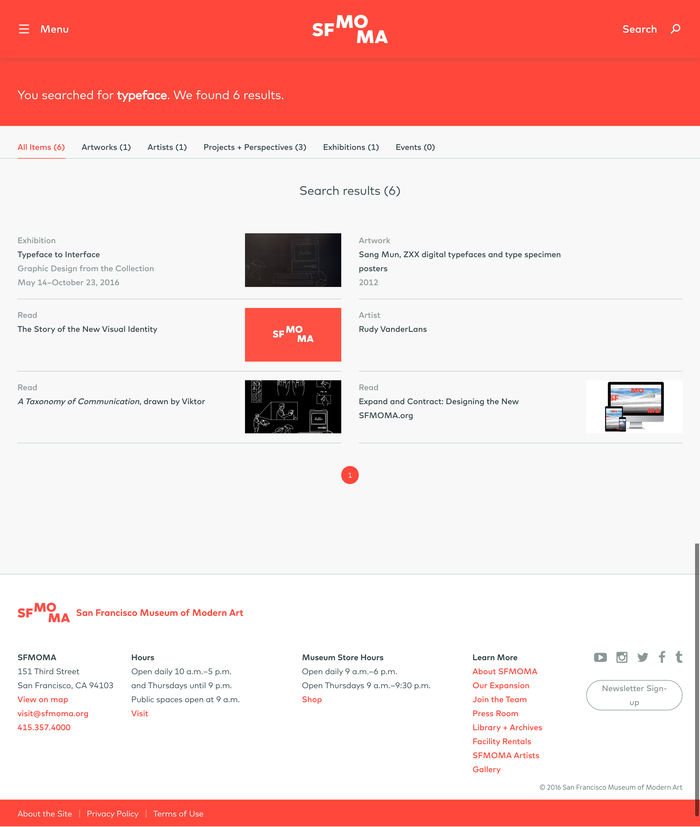This image shows a screen from the SFMOMA (San Francisco Museum of Modern Art) website. At the top, the white text displays "SF" below "MO" and beside "MA" to the right. On the left side, there is a menu button represented by three lines, and on the right is a search bar with the text "Search for typeface" in white.

The interface reveals that six results were found. A breakdown of the results includes: 
- All items (6)
- Artwork (1)
- Artist (1)
- Projects and Perspectives (3)
- Exhibit (1)
- Events (none)

One highlighted result titled "Typeface to Interface" shows various categorized results, including an artwork from 2012 titled "The Story of the New Visual Identity" by artist Rudy VanderLans. Another highlighted result is "Road: A Transition of Communication."

At the bottom, the screen provides details about SFMOMA's location at 151 3rd Street, San Francisco, California 94103, with a "View on map" button. Contact information includes an email address and a phone number, followed by the museum's operating hours.